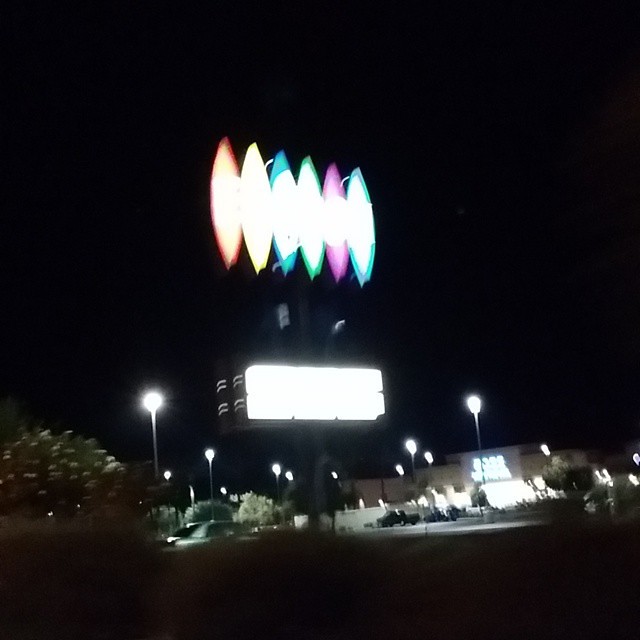This is a color photograph taken at night depicting a blurry image of a storefront or a business area, with the scene framed by a dark sky. The focal point is a large, illuminated sign in the center, mounted on a tall pole approximately 30 feet high. The sign has two parts: a glowing white rectangular section at the bottom and a series of multicolored, oblong diamond shapes on top, which include shades of red, yellow, blue, green, pink, and teal. The lights are blown out and blur the shapes, making the exact details difficult to discern.

In the foreground, there are additional illuminated objects, including what appear to be streetlight heads scattered throughout the parking lot area, contributing to the bright, hazy atmosphere. To the left of the sign, some vegetation, possibly shrubs, can be seen. The background reveals the silhouette of a building to the right, which also has a lighted sign, though its details are indiscernible. The entire scene is characterized by the interplay of various lights against the pitch-black night sky.